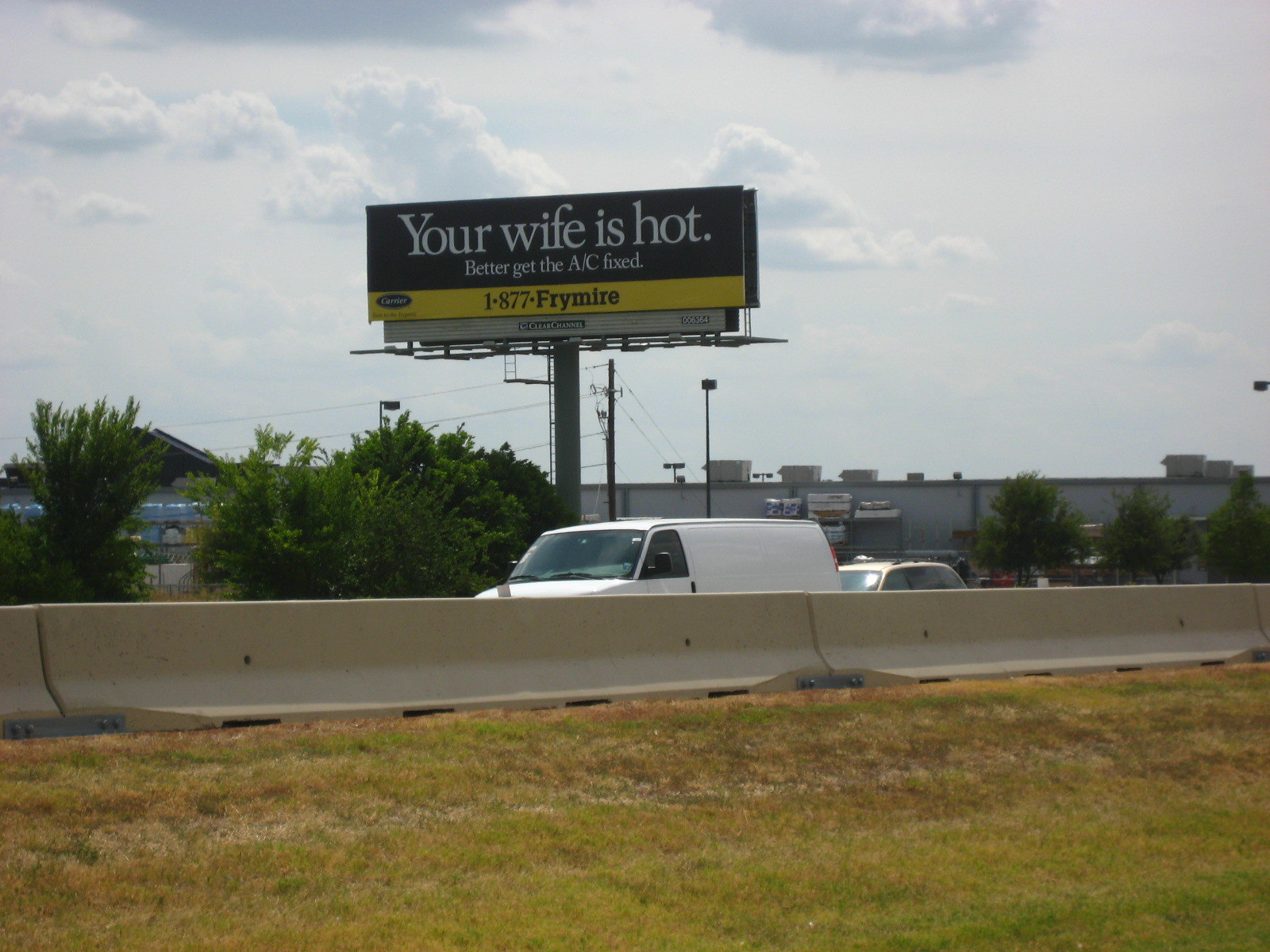This color photograph captures a busy highway scene on an overcast day, with the sky filled with gray, fluffy clouds. The foreground features a grassy median with some patches turning yellow and brown, bordered by concrete barriers and culverts stretching horizontally. Dominating the scene is a prominent billboard with a black background and white lettering that humorously reads, "Your wife is hot. Better get the AC fixed. 1-877-FRYMEYER." A white van, likely a Dodge, drives in the left lane, while a smaller car follows in the right lane. To the right of the highway, there are lush green trees and a towering building with visible air conditioning units on its roof, suggesting an industrial area. The billboard is supported by a metal pole and is flanked by two large bushes. Notably, no people or animals are visible in the image.